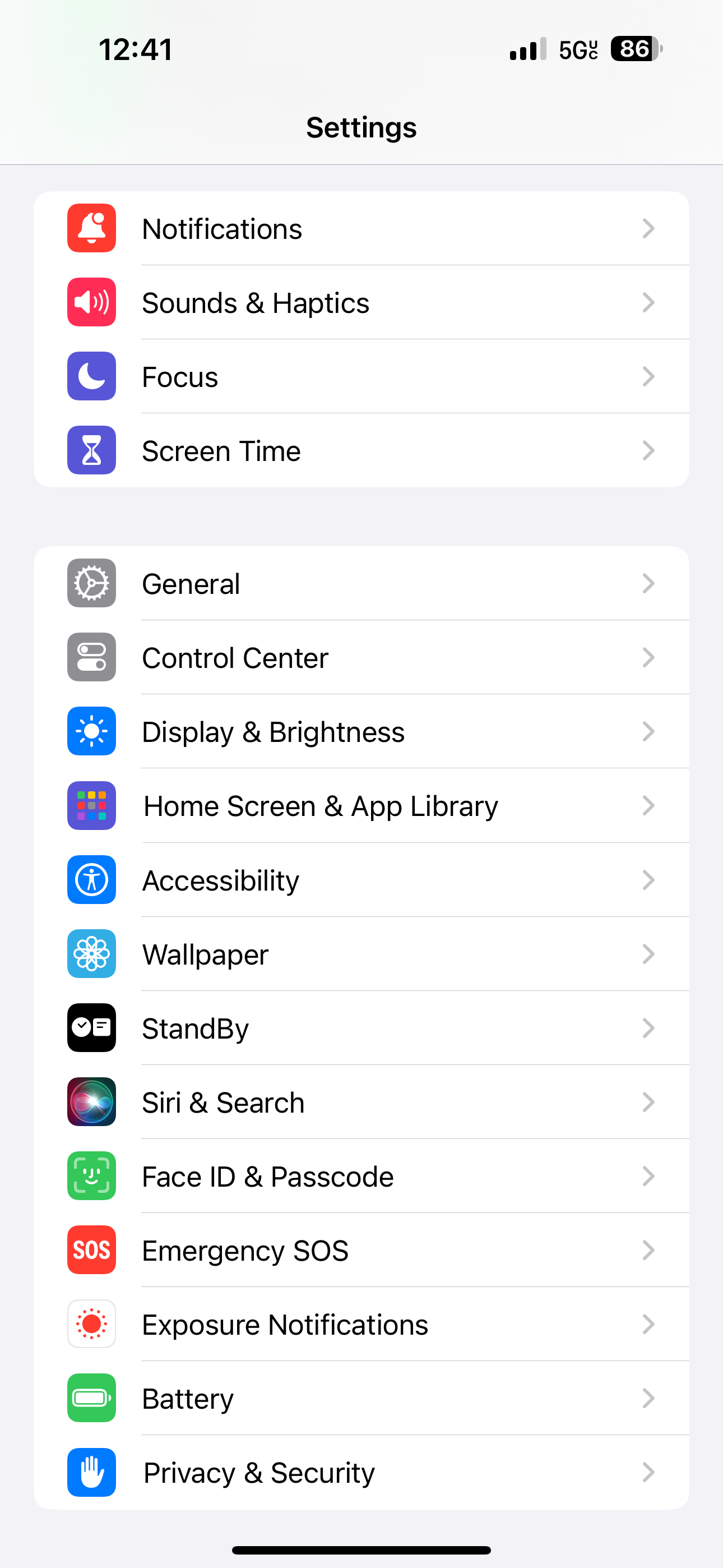The image depicts a digital interface with a light blue background, showcasing the "Settings" menu of a device. At the top of the screen, the time is displayed as "12:41," accompanied by a "5G" network indicator. The "Settings" header stands prominently at the top.

Below the header, the interface is divided into several white rectangular sections, each containing different settings categories:

1. The first section includes:
   - Notifications
   - Sounds & Haptics
   - Focus
   - Screen Time

   Each category is separated by thin lines and has a right-pointing arrow at the end.

2. The second section features:
   - General
   - Control Center
   - Display & Brightness
   - Home Screen & App Library

   The "Home Screen & App Library" option appears to be highlighted. Similar to the previous section, each category is separated by lines and includes a right-pointing arrow.

3. The third section contains:
   - Accessibility
   - Wallpaper
   - Standby

   All options within this section also have right-pointing arrows.

4. The fourth and final section lists:
   - Siri & Search
   - Face ID & Passcode
   - Emergency SOS
   - Exposure Notifications
   - Battery
   - Privacy & Security

   Each of these categories is marked with a right-pointing arrow.

At the bottom of the screen, there is a distinct black line stretching across the width of the display. The entire interface is unified by the light blue background, offering a clean and organized appearance indicative of the device's "Settings" menu.